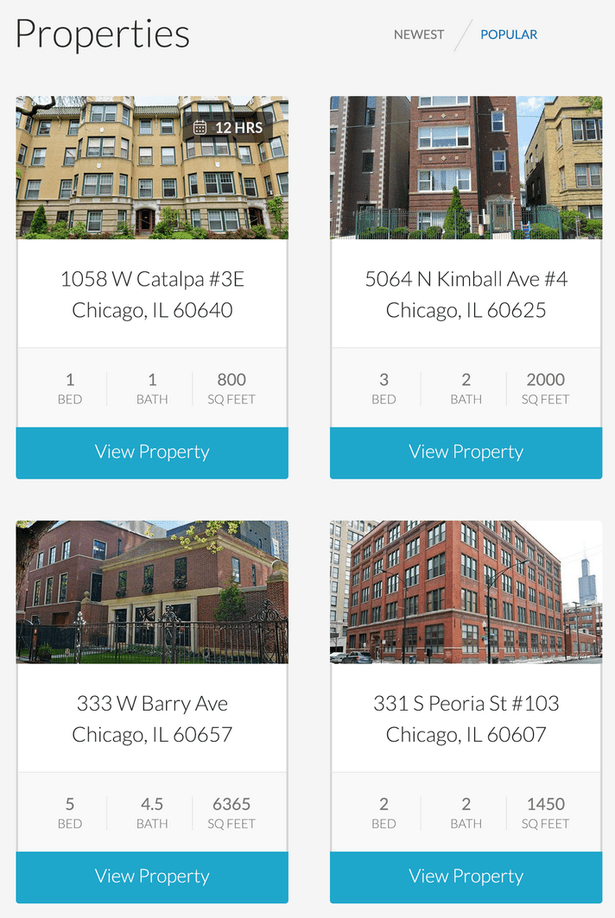The webpage showcases a selection of properties available for viewing. At the top, the header "Properties" is prominently displayed, with a sorting option on the right labeled "Newest/Popular." 

The first listing features a contemporary, four-story apartment complex with clean, earth-toned aesthetics. The address is 1058 West Catalpa, Unit 3 East, Chicago, Illinois, 60640. This property offers one bedroom, one bathroom, and spans 800 square feet. A blue "View Property" button is available for more details.

Next, to the right, is a traditional red-brick apartment building with at least four visible stories, possibly more. The background showcases a clear blue sky and some greenery, with the building enclosed by a fence. The address for this property is 5064 North Kimball Avenue, Unit 4, Chicago, Illinois, 60625. It includes three bedrooms, two bathrooms, and encompasses 2,000 square feet. There is also a blue "View Property" button for further information.

On the lower left-hand side, the third image shows a mix of two- and three-story brick buildings with wrought iron fencing. Some greenery is visible. The address here is 333 Westbury Avenue, Chicago, Illinois, 60657. This spacious property includes five bedrooms, four and a half bathrooms, and an expansive 6,365 square feet. A blue "View Property" button is available to explore more about this listing.

To the right of this, the final image shows a large, cube-like brick apartment complex with five floors situated in an inner-city setting that lacks greenery. Streetlights are visible in front. The address is 331 South Peoria Street, Unit 103, Chicago, Illinois, 60607. This property features two bedrooms, two bathrooms, and covers 1,450 square feet. Like the other listings, a blue "View Property" button is provided for additional details.